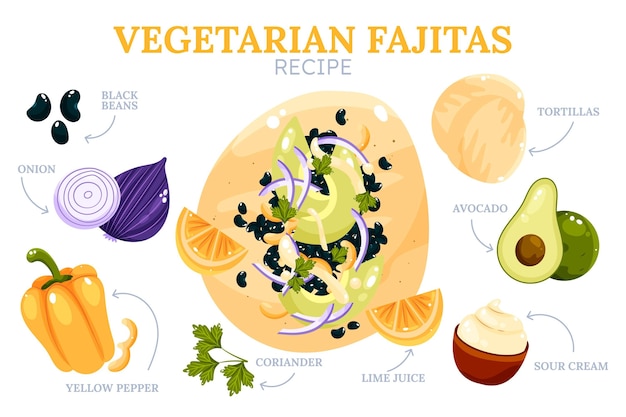This visually engaging banner, primarily designed in a portrait perspective slightly wider than it is tall, serves as a recipe guide for Vegetarian Fajitas. At the top, the title "VEGETARIAN FAJITAS" is prominently displayed in centered, orangey-yellow capital letters, followed by the word "RECIPE" in a smaller, light-medium gray, centered font. The collage-like illustration on a plain white background features various colorful ingredients identified with arrows pointing to their respective images. Starting from the upper left, there are black beans, followed by onions, yellow peppers, and tomatoes. On the right-hand side, upper right corner, two tortillas are laid flat. Moving downwards beneath the central tortilla, there are coriander and a label for lime juice, which visually depicts orange slices. The lower right area showcases a small bowl of sour cream and a halved avocado displaying its pit. At the very center of the image, an illustration of a completed fajita showcases all these ingredients spread on a flat tortilla, collectively creating a visual recipe guide. Despite the mixed styles of clip art used, the image effectively conveys the necessary elements for making delicious vegetarian fajitas.